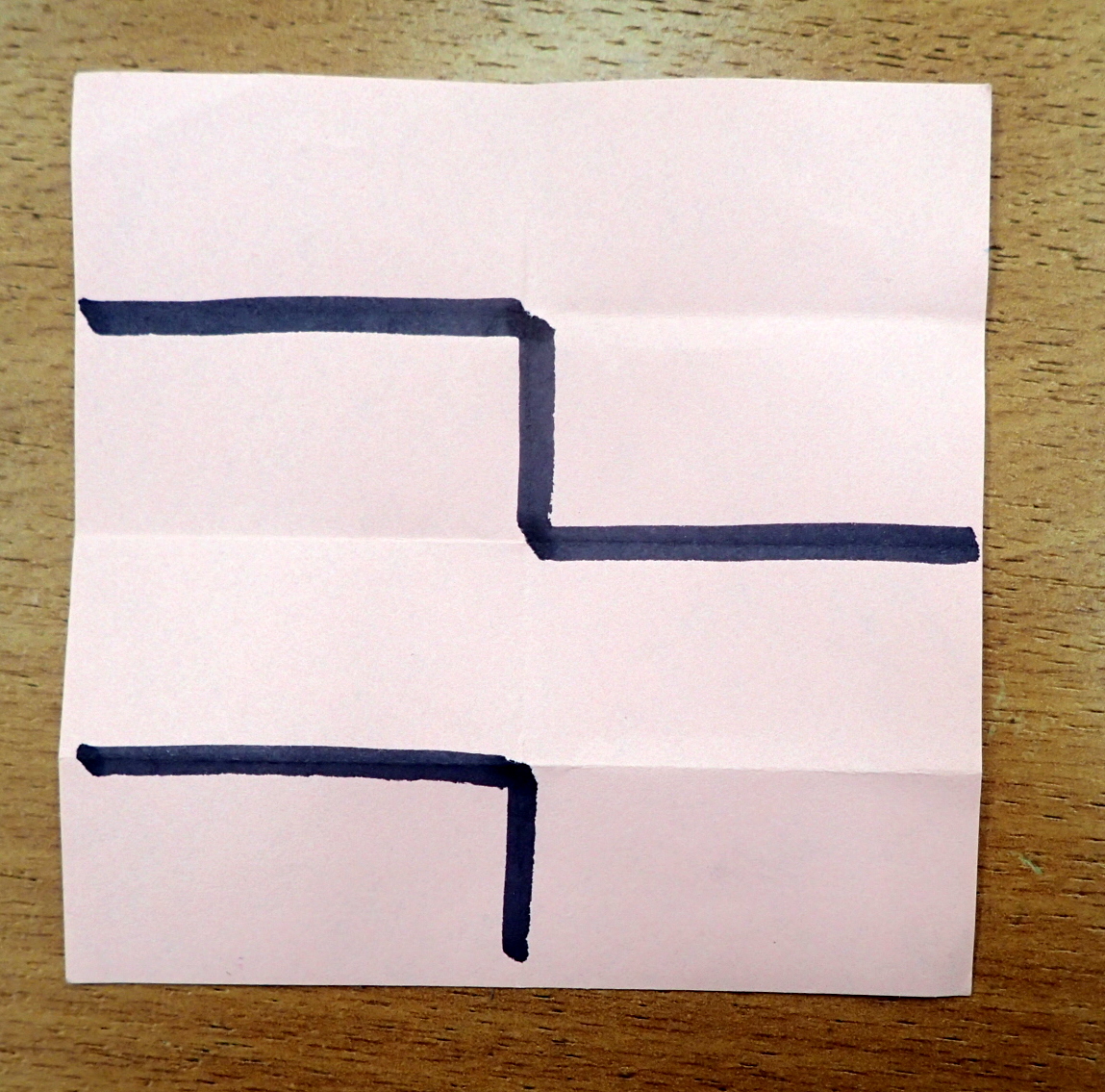A pink post-it note, folded into three sections, is placed atop a brown, wooden surface, captured in fine detail. The wooden background shows a gradient of light, with a lighter spot in the center, transitioning to darker brown on the left and right, revealing the wood grain running horizontally across the image. The post-it note features two squiggly lines: the first starts towards the middle, dips down, and then veers to the right, while the second line goes straight to the middle before sharply descending. The table, likely a laminated wood or particle board with visible finishing, supports the note prominently, highlighting its texture and the distinct folds dividing the note into bottom fourth, middle, and top fourth sections.